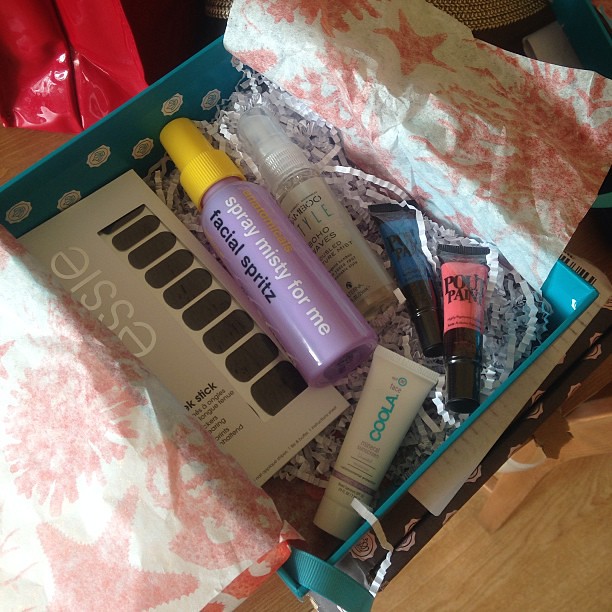The image showcases a detailed view of a cosmetics gift box or subscription box set against a rustic wooden floor. The border of the rectangular box is blue, and it is adorned with red and white tissue paper that appears to cover the bottom and extends out over the sides, sporting a star or floral pattern. Seemingly cushioning the cosmetic products are strips of shredded accordion paper.

In the upper left corner of the image, there's a glossy red bag, adding a vibrant accent to the scene. The contents of the box include a variety of cosmetics, predominantly featuring several tubes and bottles. Centered in the box is a prominent purple tube with a yellow cap labeled "Anatomicals Spray Misty for Me Facial Spritz." Below it, pointing towards the lower left corner, is a white tube marked "Coola" in light blue print. Above this, there are two additional small tubes; one is pink with a black top, and the other is blue with a black top.

To the right of the purple tube is another slightly smaller white tube with a white top. In the upper left corner inside the box is a small rectangular package labeled "Essie" on a beige background, alongside smaller brown rectangles that create a pattern. The entire arrangement and presentation of the box and its contents make it the centerpiece of the photograph.